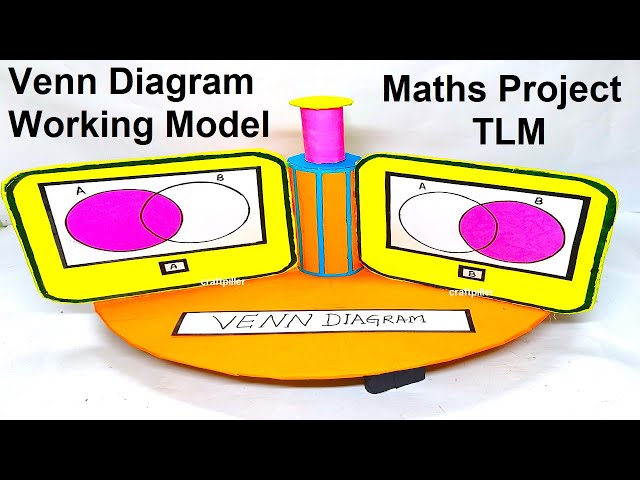The image depicts a vibrant and detailed illustration of a Venn diagram model, seemingly captured from a video, as suggested by the black bars at the top and bottom of the image, which are typical of screenshots that do not fit the screen properly. The top left corner of the image features the text "Venn Diagram Working Model," while the top right corner reads "Maths Project TLM," both in black text on a white background.

Central to the image is an orange circular platform, described as an orange turntable or cylindrical board. This platform prominently displays the words "Venn Diagram" in black letters on a white background. Positioned on either side of a central cylindrical pillar, which appears to have pink and yellow components, are two signs or screens.

Each screen showcases an example of a Venn diagram labeled as Exhibit A and Exhibit B. Both screens are designed with a yellow round rectangle as the border and a white rectangle within it. Exhibit A, on the left, displays a Venn diagram where the left circle is entirely filled with magenta, while the right circle is white except for the magenta overlap. Conversely, Exhibit B, on the right, shows the right circle completely in magenta and the left circle white except for the overlapping area. This intricate model is a part of a maths project and serves as an educational tool for understanding Venn diagrams.